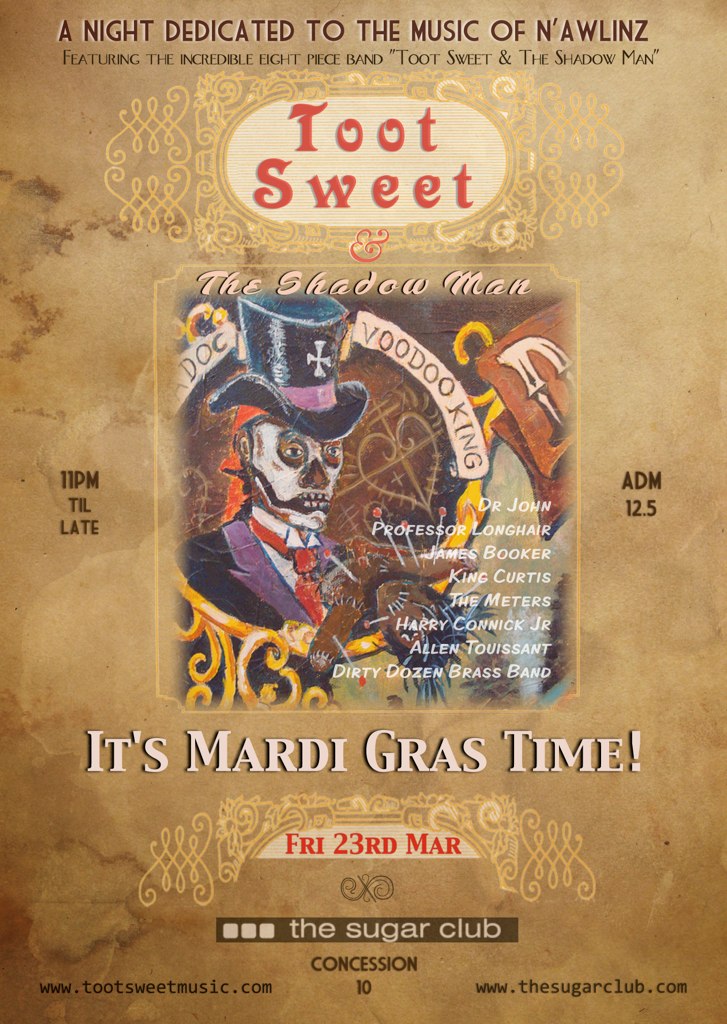This vibrant poster, illustrating a Mardi Gras event at the Sugar Club, is set against a vintage beige background. At the top, bold black text announces "A Night Dedicated to the Music of N.A.W.L.I.N.Z," followed by the subtext, "featuring the incredible 8-piece band Toot Sweet and the Shadow Man." Dominating the design is a large, ornate oval with the band name "Toot Sweet" in red, vintage typography accented with gold filigree. Below it, in a prominent square graphic, is a vivid cartoon of the Shadow Man—a skeleton figure decked out in a black top hat, purple-trimmed black coat, and red tie. The hat bears inscriptions like "Doc Voodoo King" and names of renowned musicians such as Dr. John, James Booker, The Meters, and Harry Connick Jr. Flanking this image are details about band members, event date, and price. Bold white text underneath the graphic exclaims "It's Mardi Gras time," followed by the event date "Friday, 23rd March" in red letters against a cream backdrop. At the bottom, "The Sugar Club" and concession details are listed, framed by brownish-tan patterns arching around the entire piece. This colorful, detailed illustration serves as both an invitation and a visual celebration of New Orleans' rich musical heritage.